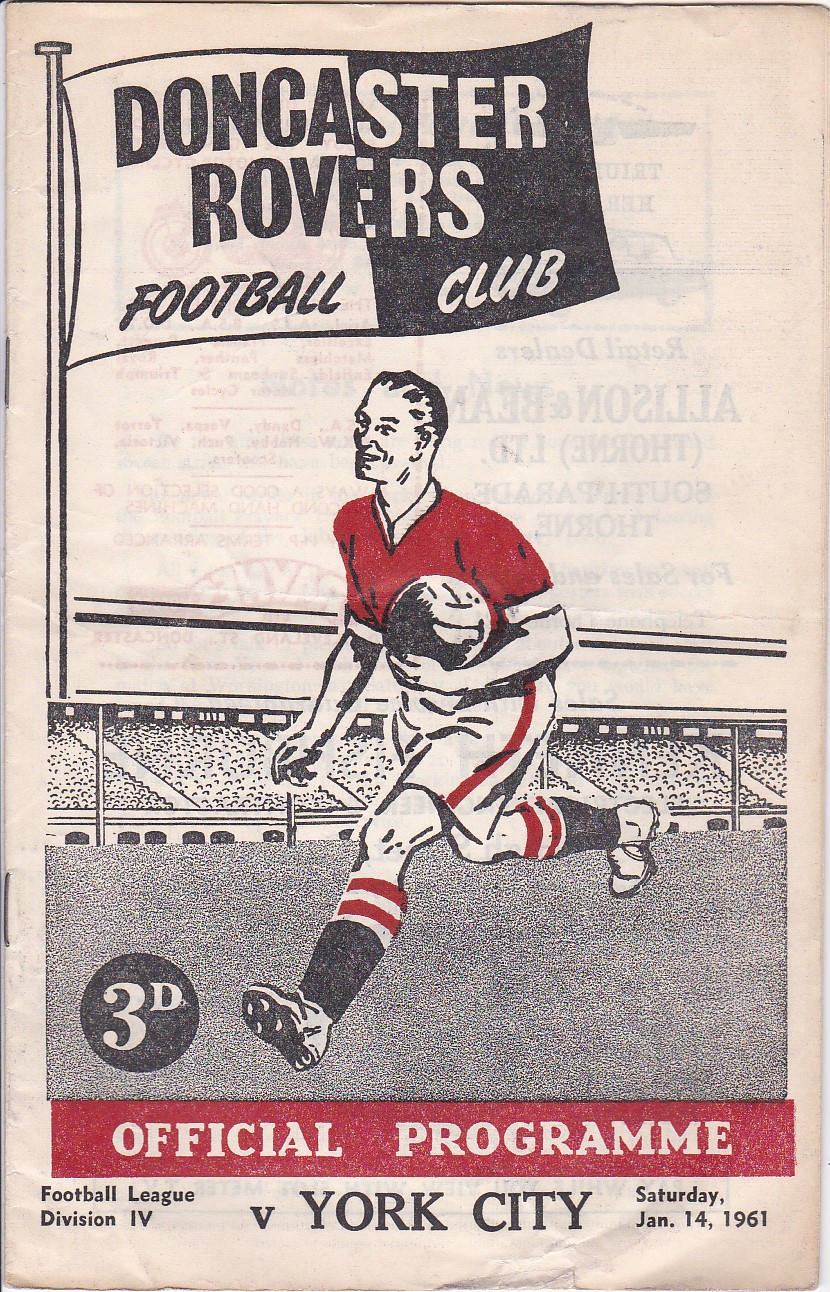The image depicts a vintage, rectangular sports-related program cover for a football match. The background is cream-colored, with illustrations primarily in black and red. Centered prominently is a dynamic drawing of a sports player, sporting a red shirt, white and red shorts, and striped black socks. The athlete, shown with short hair, is in mid-motion, holding a soccer ball and running, with both feet off the ground. Behind him is a detailed depiction of a stadium, filled with small dots representing the crowd.

In the upper left corner, a large flag reads "Doncaster Rovers Football Club," illustrated with a split black-and-white design. Below this flag, there's a red horizontal strip displaying the text "Official Program" in white. At the bottom of the poster, smaller black type provides details about the event: "Football League Division IV, V, York City, Saturday, January 14th, 1961." Additionally, a black circle on the lower left side notes the price as "3D." The entire cover appears to be an old-fashioned paper program, complete with visible staples on the left-hand side, further emphasizing its vintage nature.